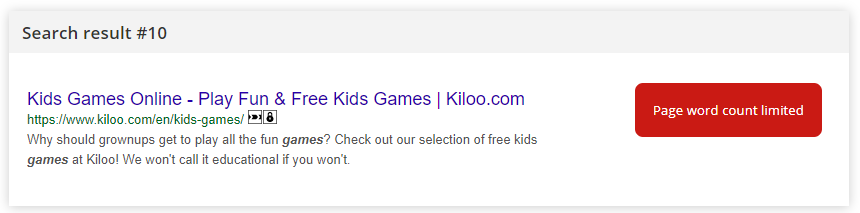The image depicts a single search result from an online search engine. At the top of the search result, within a grayish-white shaded box, the text "Search Result Number 10" is clearly displayed. Just below, in a contrasting white box, the clickable link is presented with the title "Kids Games Online - Play Fun and Free Kids Games at Killo.com." This title is highlighted in a bluish-purple font, making it stand out against the white background.

Beneath this title, the website URL "www.killo.com" is formatted in a green font, providing a visual distinction from other textual elements. The link is immediately followed by a brief description in a dark gray, almost black font, which reads: "Why should grown-ups get to play all the fun games? Check out our selection of free kids games at Killo. We won't call it educational if you won't."

To the right of this text, a red box containing the phrase "Page Word Count Limited" emphasizes a constraint on the content shown. The overall layout is minimalistic and straightforward, focusing solely on delivering essential information without distractions.